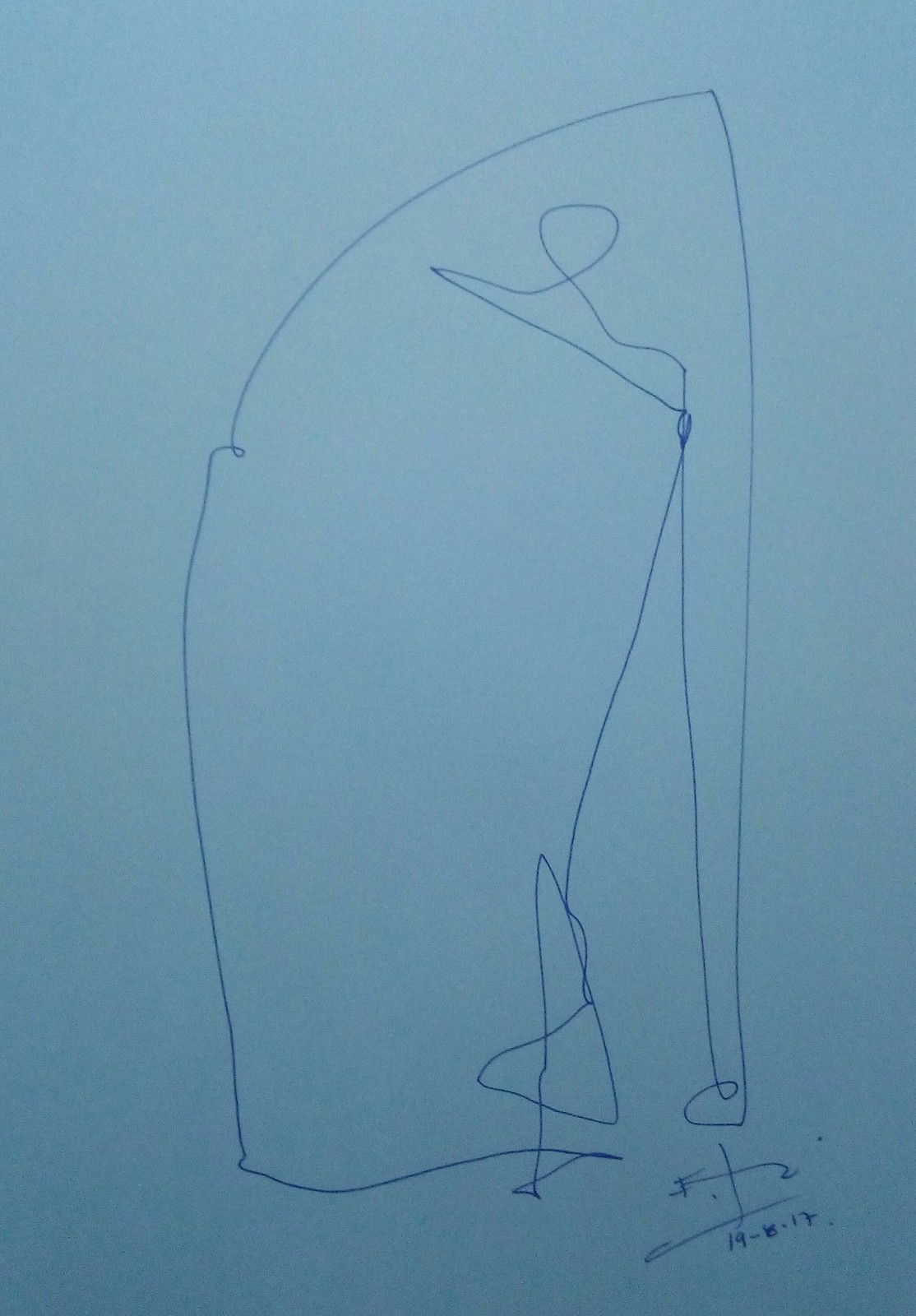The artwork is a minimalist, line-drawn piece on a rectangular sheet of paper, the proportions of which are twice as long on the sides compared to the top and bottom. The paper appears light gray due to the low ambient lighting, with the bottom right corner enveloped in shadows, making it significantly darker than the rest of the piece. The central figure of the drawing is a conical shape with a flat base and an almost pointed top, drawn in blue ink. This conical form inclines slightly to the right, with the pointed tip aiming toward the top right corner while the flat bottom aligns closer to the center. Notably, there is a distinguishing 'A' shape integrated into the bottom right section of the cone, and an arm-like extension from the top of the cone terminates in a rounded, foot-like shape. Below this foot shape, the artist's signature is visible, reading "FTZ" along with the date "19-8-17."